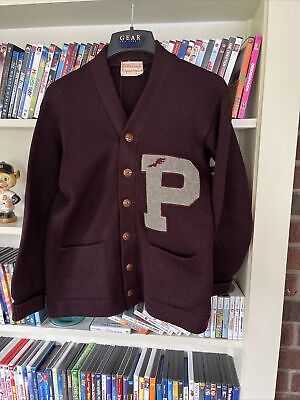In the image, there is a dark maroon or deep purple cardigan that resembles a vintage letterman's jacket. The cardigan is buttoned up with six goldish-bronze buttons and features two front pockets. It also prominently displays a large, light-colored "P" stitched onto the left breast area. The cardigan hangs from a black hanger with a silver hook, which has the word "gear" written on it, and it is hanging from the top of a white bookshelf. The bookshelf is filled with various DVDs, video game cases, and other items, including a bear statue adorned in baseball gear situated to the left of the cardigan. Below the cardigan on the next shelves are more DVDs and game cases, and additional bobblehead figures or other decorative pieces can be seen among the items on the shelves.